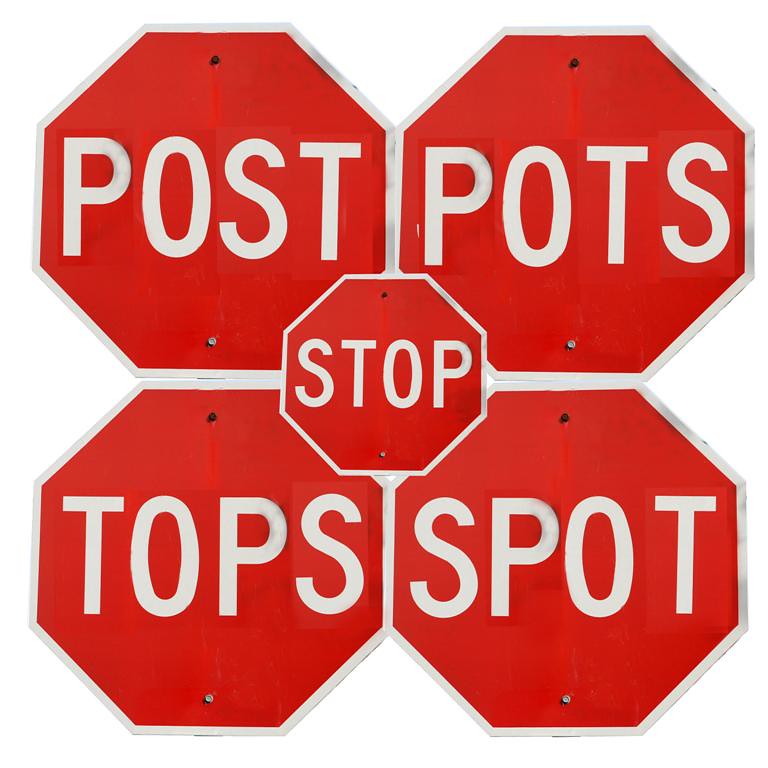This photograph features a unique arrangement of five octagonal red stop signs with white trim and lettering, creating a visually intriguing pattern. Four larger stop signs are positioned to form a square, touching each other at the edges, resembling the petals of a flower around a central sign. The top left sign reads "POST," the top right reads "POTS," the bottom left reads "TOPS," and the bottom right reads "SPOT." In the center of these four larger signs is a smaller stop sign that correctly spells "STOP." The signs are connected by a silver rim and superimposed on a plain white background, giving a clear view of the screws holding them in place, which are dark brown and silvery in color. The white background further highlights the striking red and white contrast of the stop signs.